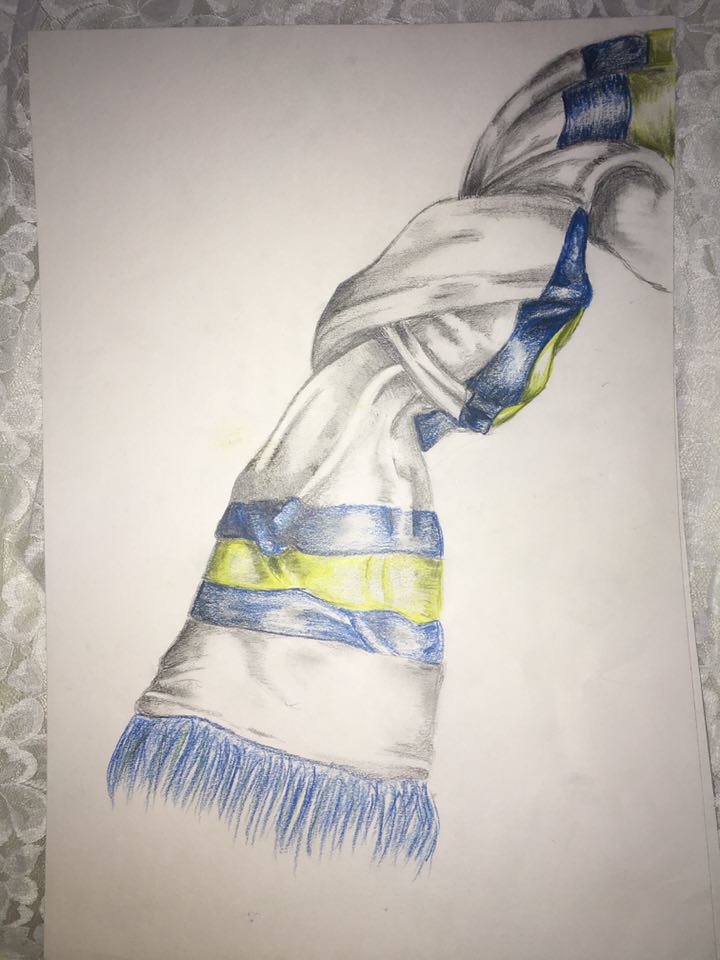This photograph showcases a meticulous piece of artwork executed on white paper, which is set against a backdrop of floral-patterned white fabric. The focal point of the drawing is a delicately knotted scarf rendered in shades of pencil, accentuated with carefully applied colored pencils. The scarf, predominantly white, is intricately shaded to create a realistic three-dimensional appearance. The knot is centrally positioned, with the fabric elegantly flowing outward from the tight center. The finishing touches of the scarf feature alternating stripes of blue and yellow, along with a blue fringe that adds a touch of vibrancy and contrast. The harmonious blending of pencil and colored pencil techniques highlights the artist's skill and attention to detail, making this piece a captivating study of texture and color interplay.